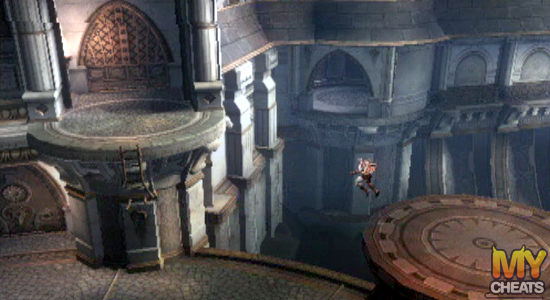This detailed image is a screenshot from a 3D platformer video game, showcasing a dynamic and adventurous scene set against the backdrop of a gothic or renaissance-styled castle. The scene captures the main character jumping from a round platform on the right-hand side to a platform on the left, crossing a significant gap that spans dozens of feet and rises about 10 feet above the lower platform. Below, there is a pathway or balcony suggesting a large drop-off, further emphasized by a broken ladder leading up to the target platform. The character appears to be equipped with brown boots and possibly carrying a weapon, indicating tactical gear.

The watermark "MY CHEATS" is prominently displayed in the bottom right corner, with "MY" in capitalized yellow letters adorned with little horns on the M's, and "CHEATS" in white letters beneath. This adds a playful yet informative touch to the image. The environment is devoid of any other characters, animals, plants, or trees, focusing entirely on the architecture and the challenge at hand. There is a large bronze-colored gear at the bottom right, adding to the intricate design elements within the game. The overall layout suggests multiple surfaces and levels within a vast, open castle exterior.